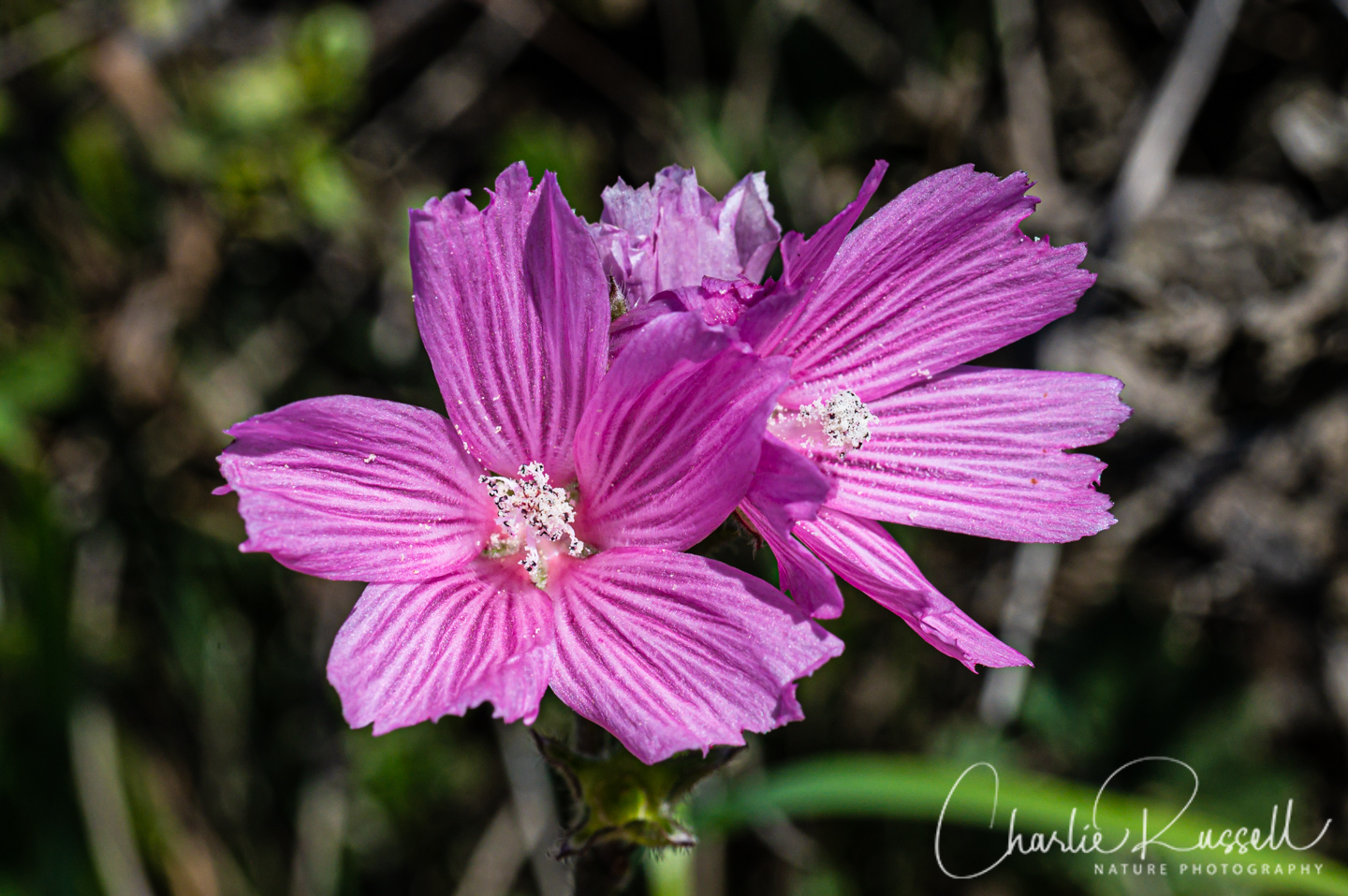This professional photograph captures a close-up of two or perhaps three purple flowers, each with approximately five petals. The flowers, showcasing shades that range from light purple or pink to darker hues at the tips, are the dominant focus of the image, displayed prominently in the center. Their petals exhibit some signs of wear, possibly from caterpillars or natural decay, while the centers bloom with intricate, short white flowery extensions accented with specks of black. The background, a blend of greens and occasional browns, appears blurred, reinforcing the flowers' prominence. At the bottom right corner, a watermark in a loopy cursive script reads "Charlie Russell," with "Nature Photography" in a smaller, more standard font beneath it. This elegant and detailed composition emphasizes the delicate beauty of the foreground flora against an indistinct yet natural backdrop.